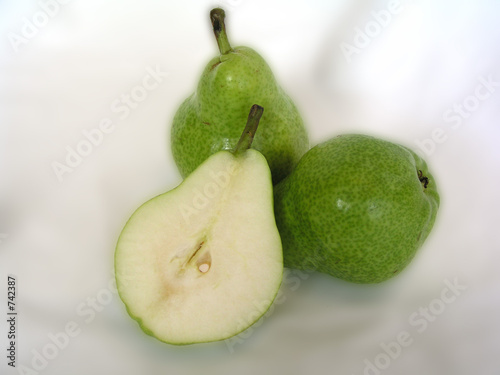The image is a detailed Adobe Stock photograph of three green pears arranged on a light gray cloth background. The composition includes two whole pears with stems, and one pear that has been sliced in half to reveal its white, seed-filled interior. One whole pear is positioned to the left, another to the right, and the halved pear is placed diagonally above the whole pears. There is a watermark that reads "Adobe Stock" along with stock number 742387, found in black text in the bottom left corner, rotated counterclockwise. This visually appealing image is presented in a clean, professional style, suitable for advertisement purposes.